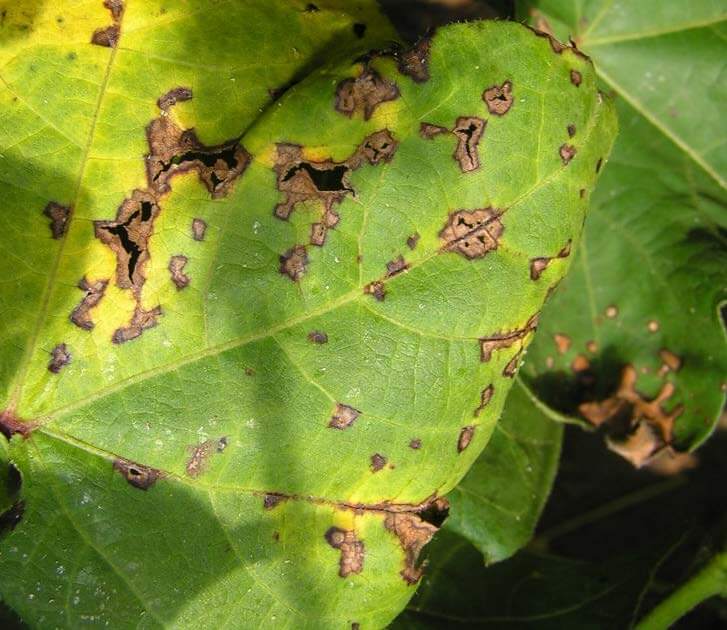This image showcases a close-up of a green leaf, likely from a tree and possibly resembling a maple leaf, with clear signs of insect activity. The prominent leaf in the foreground is almost equal in length and width, featuring various bite marks and small, brown spots caused by bugs munching on it. These round holes and brown discolorations suggest insect damage, potentially from aphids, which are tiny mites known to harm plants. The scene is set outdoors, where the primary leaf exhibits yellowish veins amidst its green surface. Surrounding this main leaf are other green leaves, one to the right also showing insect bites and a notable black spot. The blurred background hints at green stems, completing the natural setting.